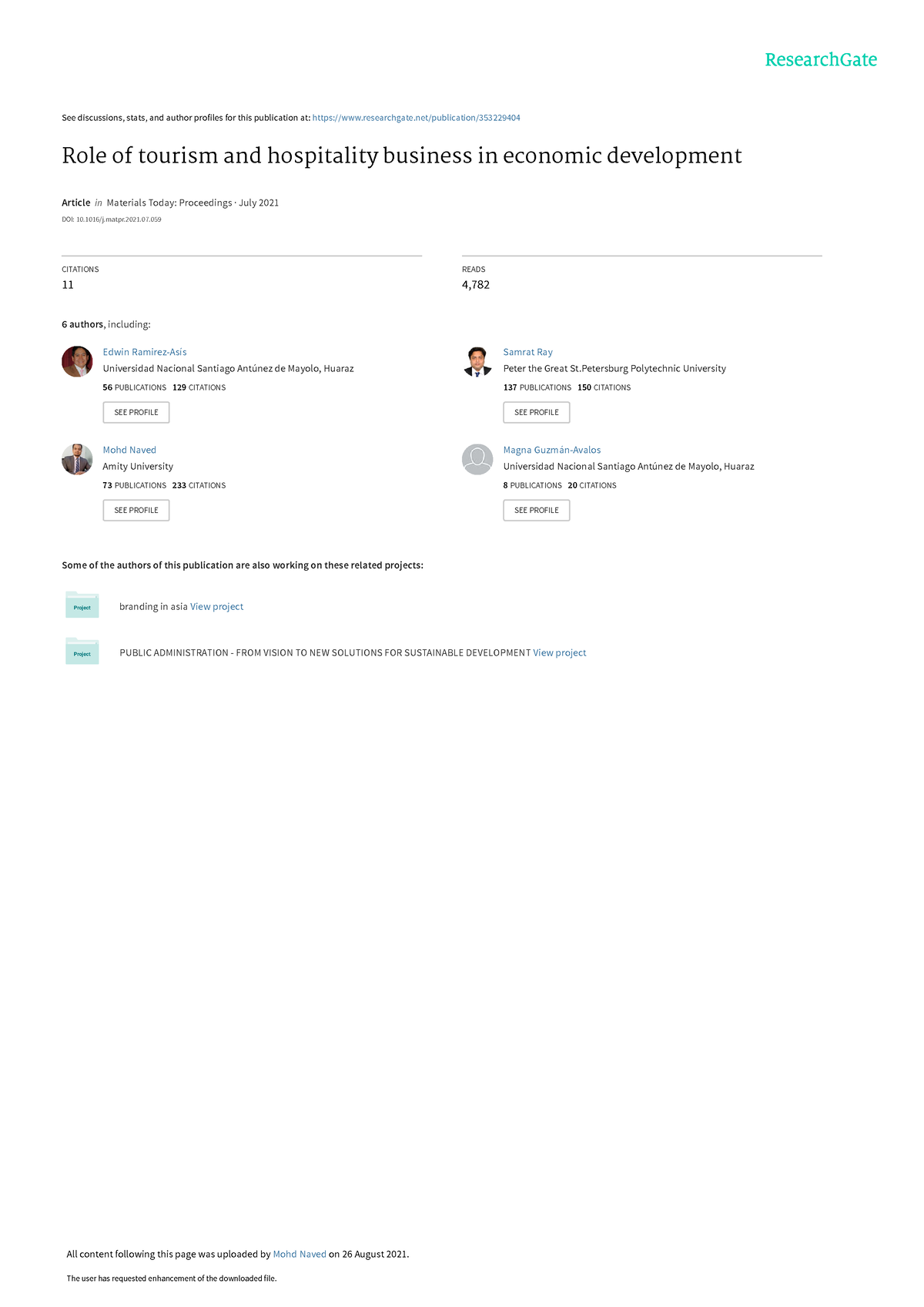The image is a screenshot from a mobile phone display, showcasing a publication summary on the ResearchGate platform. The top right corner features the ResearchGate logo in green. Beneath the logo, in very small print, it reads: "See discussions, stats, and author policies for this publication at" followed by a clickable link. The title of the publication is prominently displayed as: "Role of Tourism and Hospitality Business in Economic Development." This article is part of the "Materials Today: Proceedings," specifically the July 2021 edition.

Further details include citation information, indicating the publication has been cited 11 times. The authors listed are: Edwin Ramirez SC, Mohad Neved, Samarat Ray, and Magna Gomez Avalos. The lower portion of the screen is predominantly white space with minimal text, adding a clean, uncluttered look to the overall layout.